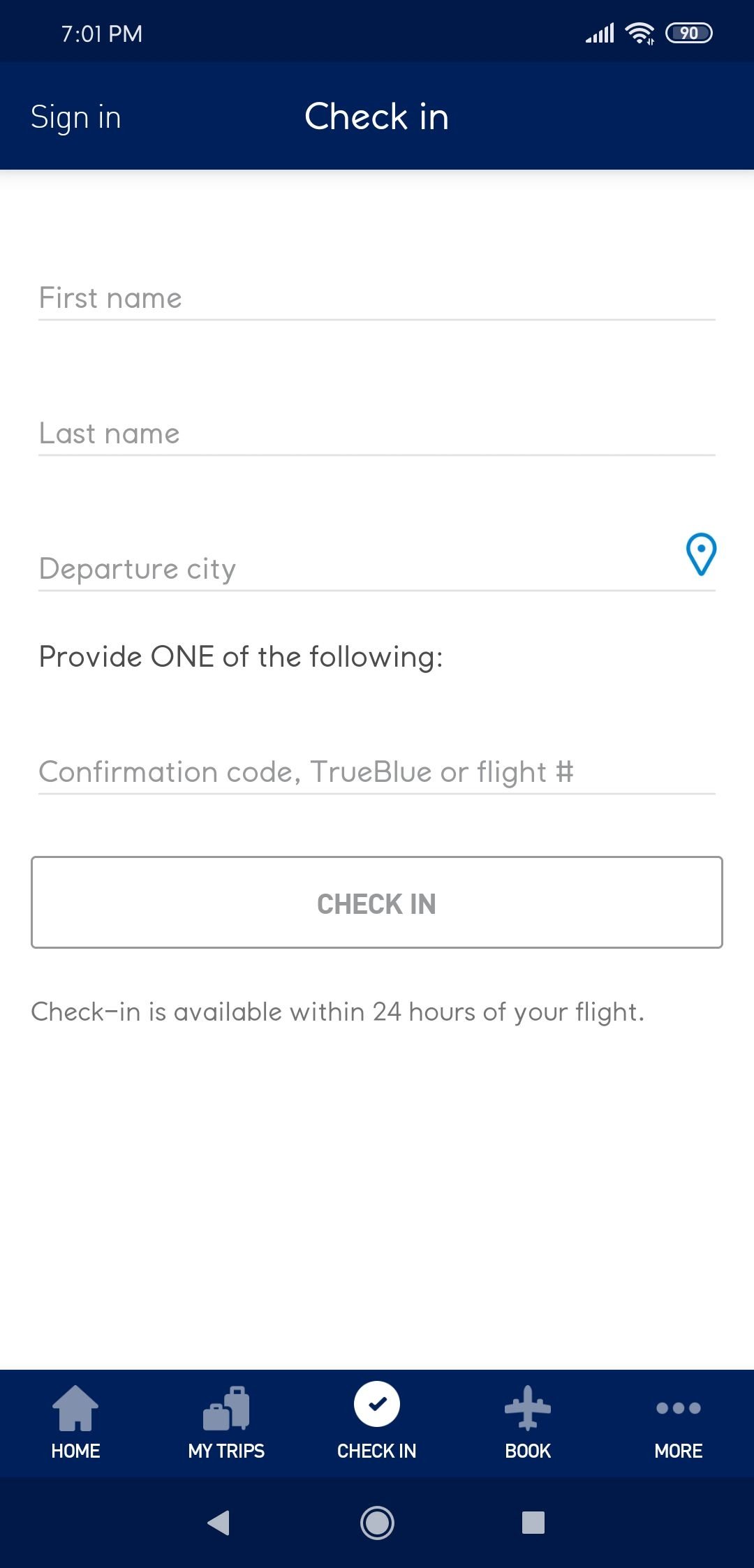This image features a check-in interface with a navy blue-themed design. The top header, set against a navy blue background, displays the time "7:01 p.m." in the top right corner, along with a battery icon indicating a 90% charge on the far right side. Below this header is a sign-in button on the left and a centered title that reads "Check-In".

The main section of the box consists of four input fields: 
1. **First Name**
2. **Last Name**
3. **Departure**
4. **Confirmation Code, TrueBlue Number, or Flight Number**

A text prompt above the confirmation code line states, "Provide one of the following." Directly beneath these input fields is a check-in button. Following this button, there is a line of instructional text informing users, "Check-in is available within 24 hours of your flight."

The bottom header, mirroring the navy blue background of the top header, contains four icons: 
1. **A house icon** for Home
2. **Two luggage bags icon** for My Trips
3. **A checkmark icon** for Check-In
4. **An airplane icon** for Book

Additionally, there are three ellipses indicating more options. The remainder of the webpage, where the input fields are situated, has a clean white background, creating a clear and user-friendly interface.